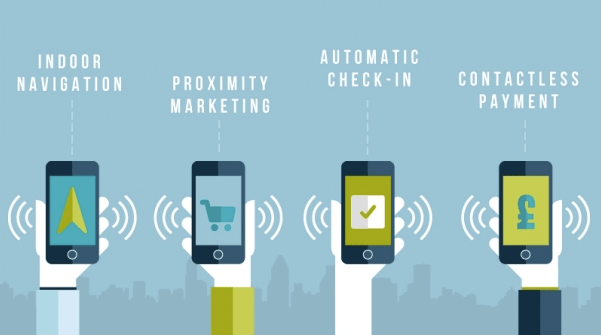The animated image features a light blue background with a silhouette of city skyscrapers at the bottom. Centered in the foreground are four identical smartphones, each held by a hand. The hands emerge from white arms wearing different colored sleeves just above the wrist. Starting from the left, the first phone, held by a hand with a blue shirt sleeve and a glimpse of a black underlayer, displays a green arrow pointing up with the caption "Indoor Navigation" in white text connected by a line. The second phone, held by a hand in a gold shirt, shows a shopping cart and has the caption "Proximity Marketing" above it. The third phone, held by a hand without a visible sleeve, displays a white box with a green checkmark, accompanied by the text "Automatic Check-in". The final phone, held by a hand in a black sleeve, features the British Pound symbol (£) on its screen with the caption "Contactless Payment" above. Each phone also has sound wave-like lines emanating from it, enhancing the impression of connectivity and interaction.